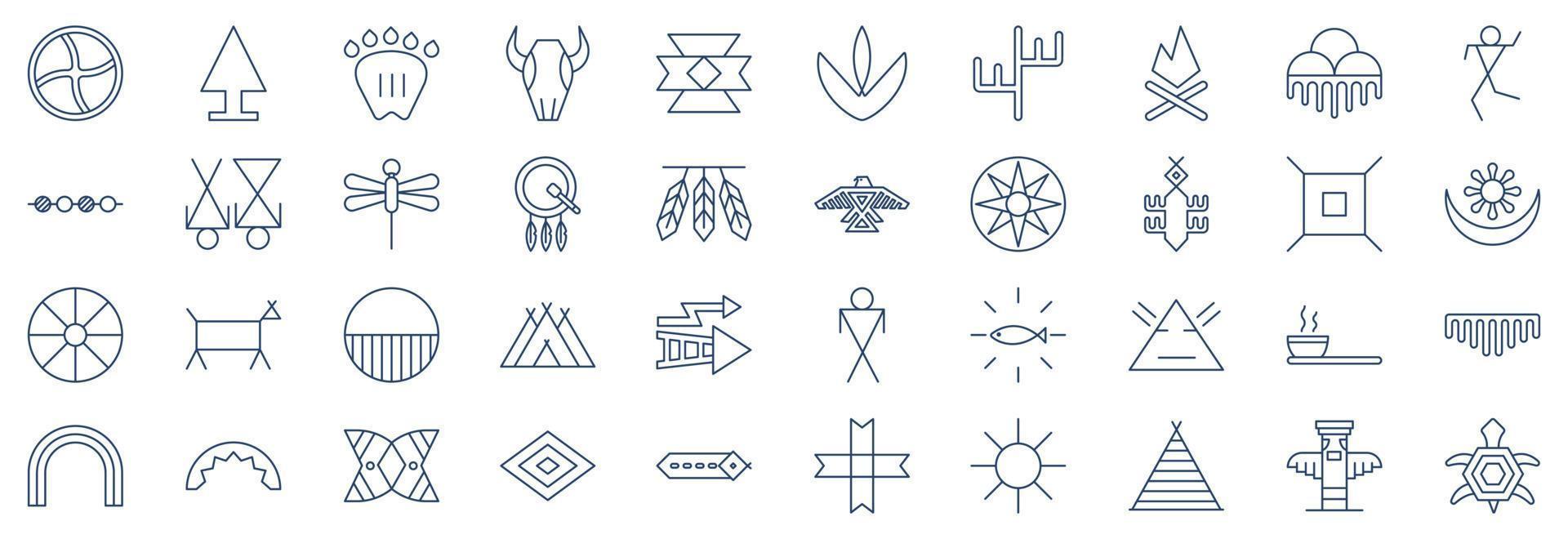The black and white image, which may also be interpreted as dark navy and white, showcases a series of four rows of intricate pictographs. Predominantly, some of the symbols are reminiscent of Native American culture. In the top row, familiar figures such as a cow skull, a bear paw, a tree resembling a pine, a cactus, and a campfire are depicted. The second row features identifiable symbols including a dreamcatcher, a firefly, a phoenix, and what appears to be a chameleon. The third row continues with symbols like a dog, a campsite setup with a tent and a person, a fish surrounded by sparkles, and a cup, be it tea or soup. The bottom row displays the sun with rays, a tortoise with a detailed hexagonal shell, a totem pole, and a teepee. Scattered throughout the image are additional symbols such as an archway with double lines, a stick figure running with an upraised left arm, and an intriguing circular figure sectioned into eight parts, all contributing to the rich tapestry of this cultural illustration.